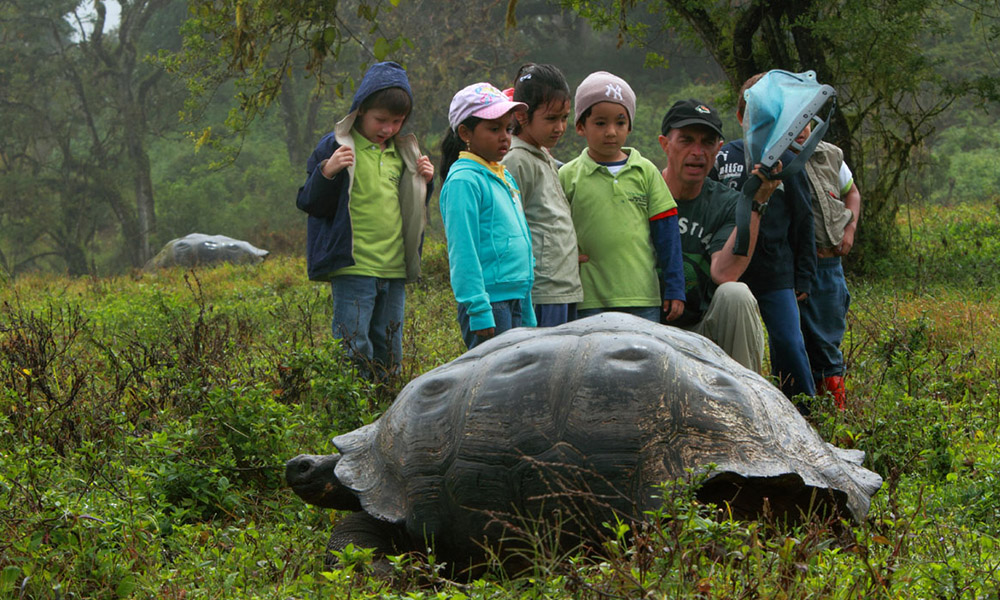In an intricate and vibrant woodland setting, a massive tortoise is the focal point of the image. Surrounding the tortoise, five young children, approximately five or six years old, stand in awe. They are dressed in long sleeves and various types of hats, which, along with the adult's attire, suggest a cool day. The man, kneeling behind the tortoise, is actively engaging the children, seemingly explaining something while holding an object that appears to be a camera. The background is rich with dense green foliage, trees, and bushes, alongside a prominent rock and a small glimpse of the sky. The children stand amidst low bushes and weeds, and another tortoise shell can be vaguely seen further back, adding a layer of depth and continuity to the scene.